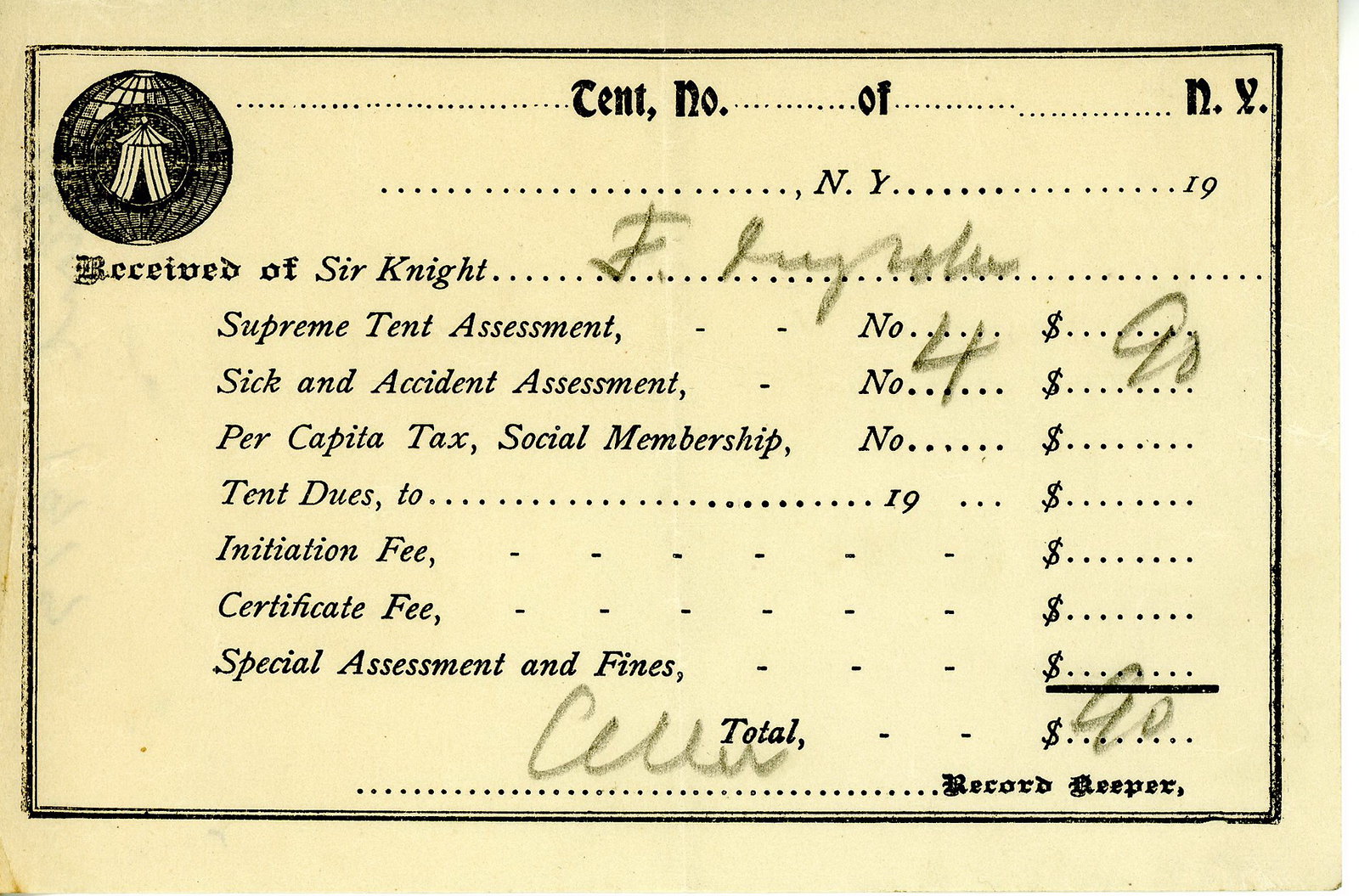The image shows an antique yellow card, potentially from the Victorian era, featuring black text. The card serves as a record-keeping document, akin to an old bill of sale or receipt, used to track various assessments and fees. In the top right corner, there is a faded black logo depicting a globe and a tent. Adjacent to this logo, there's a dotted line labeled "tent number," followed by blanks for "blank of blank, blank, New York." Below that, another dotted line reads "New York, blank, 19--."

The card's main text begins with "Received of Sir Knight," followed by an illegible handwritten name that seems to start with "F." The card enumerates various charges, including "Supreme Tent Assessment," "Sick and Accident Assessment," with the number 4 and amount 90, "Per Capita Tax," "Social Membership," "Tent Dues," "Initiation Fee," "Certificate Fee," and "Special Assessment and Fines." Most categories are not filled out except for the Sick and Accident Assessment. The total recorded is $90. The document is signed by the record keeper, with a barely legible name that appears to be "Seller."